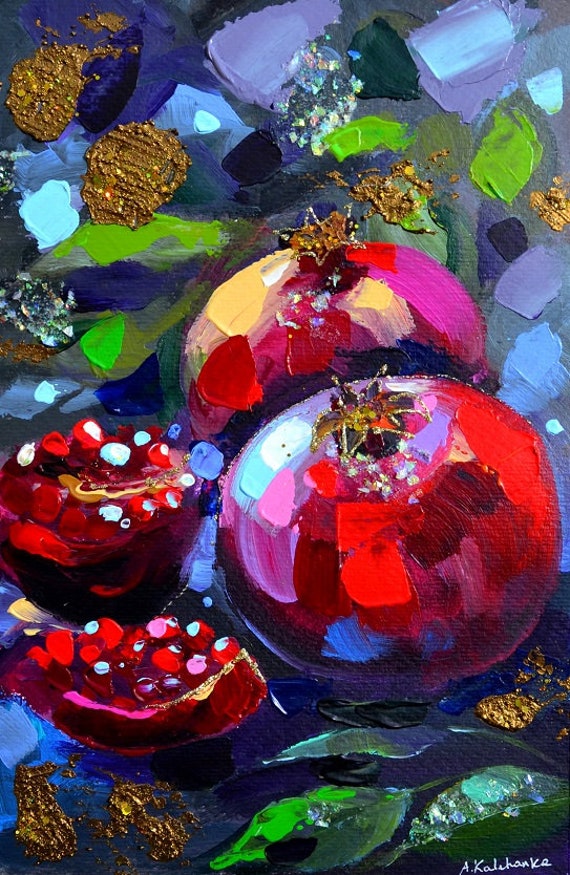This abstract, impressionist painting by artist A. Kalikahanka presents an evocative arrangement of vibrant colors and jeweled objects. Central to the composition are two richly red pomegranates with expressive brushstrokes that create small patches of white and pink, giving the appearance of a jewel-like texture. Beside them, pieces of the fruit are depicted, their segmented seeds highlighted with a bright, almost illuminating white. Scattered around the painting are various abstract shapes and colors, including green encrusted gems in the front right, gold smudges in multiple corners, and what appear to be cherries or additional jewels within a red velvet bag to the left of the pomegranates. The dark blue background contrasts strikingly with the reds, greens, and golds, enhancing the overall vividness of the painting. Despite its abstract nature, the depiction of the pomegranates and accompanying elements bursts forth with a jewel-like brilliance, blending impressionist and abstract techniques to create a detailed and captivating visual narrative.